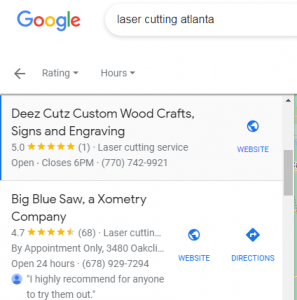This image depicts the results of a Google search carried out on a smartphone, with the user looking for laser cutting services in Atlanta. At the top, the screen displays a 'back' button, user ratings, and business hours, suggesting that the user has delved deeper into the search results.

The first result listed is "DEEZ Cuts" which offers custom woodcrafts, signs, and engravings. This business boasts a five-star rating. The listing includes a category indicating it is a laser cutting service, with operational hours listed as closing at 6 PM. The contact number given is 770-742-9921, and there is an icon and link for the business's website on the right side of the entry.

The second result is "Big Blue Saw," a company specializing in geometry-related services. It holds a 4.7-star rating based on 68 reviews and offers laser cutting services by appointment only. It is noted to be open 24 hours. The provided contact number is 678-929-7294. Additionally, there is a quote from a user who "highly recommends anyone to try them out.” Next to this quote, there is a small profile icon, depicted as a simple blue silhouette of a generic head and shoulders within a light circle. To the right of the quote, there are options for visiting the website and getting directions.

This image provides a snapshot of the detailed information available on Google search results, highlighting customer ratings, contact information, operational hours, and additional options for further engagement with the businesses listed.